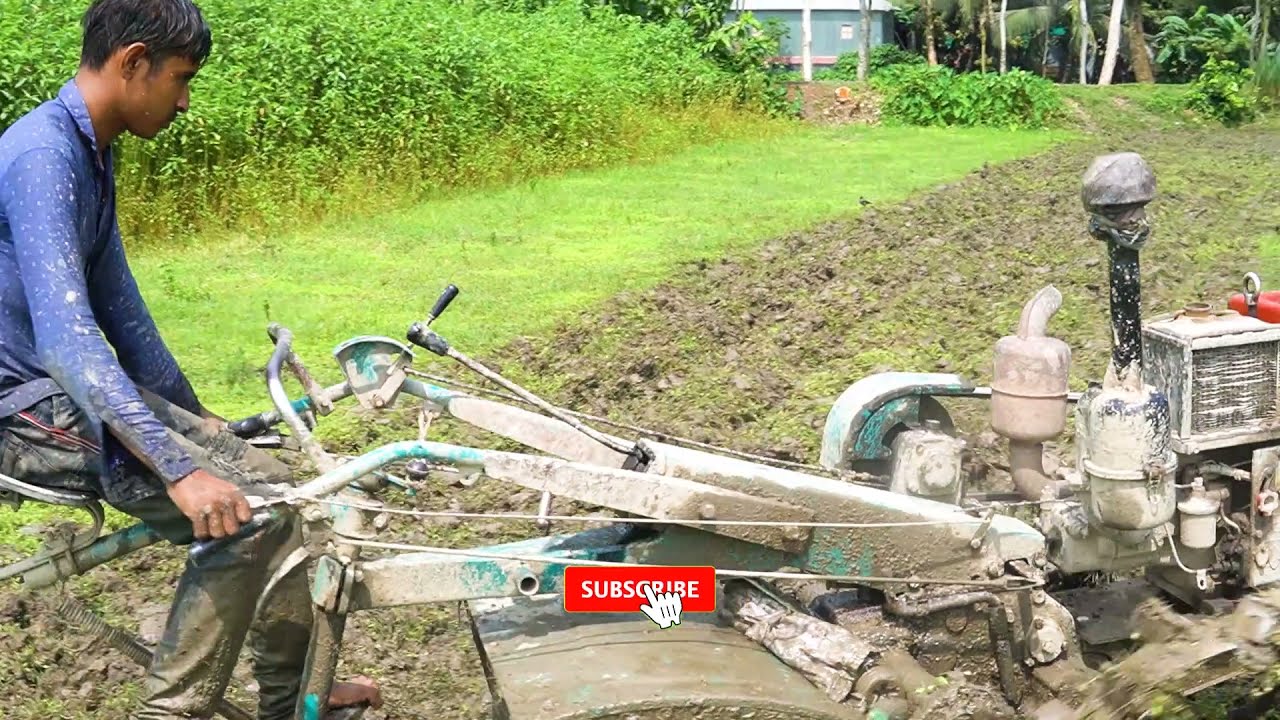In the daytime outdoor scene, a young man of East Indian heritage, wearing a long-sleeved blue shirt splattered with dirt and mud, is operating a large tiller machine. The tiller is caked with wet soil and some paint, featuring various attachments and a chain. The man, who has short black hair, seems to be preparing the land for planting. The field, which is partially tilled, has green grass and bushy vegetation on the left side, extending diagonally across the frame. In the background, there is a path, a stand of trees, and a blue building located around a hundred to two hundred feet away. The expansive field shows no current growth, indicating it's in the early stages of cultivation.